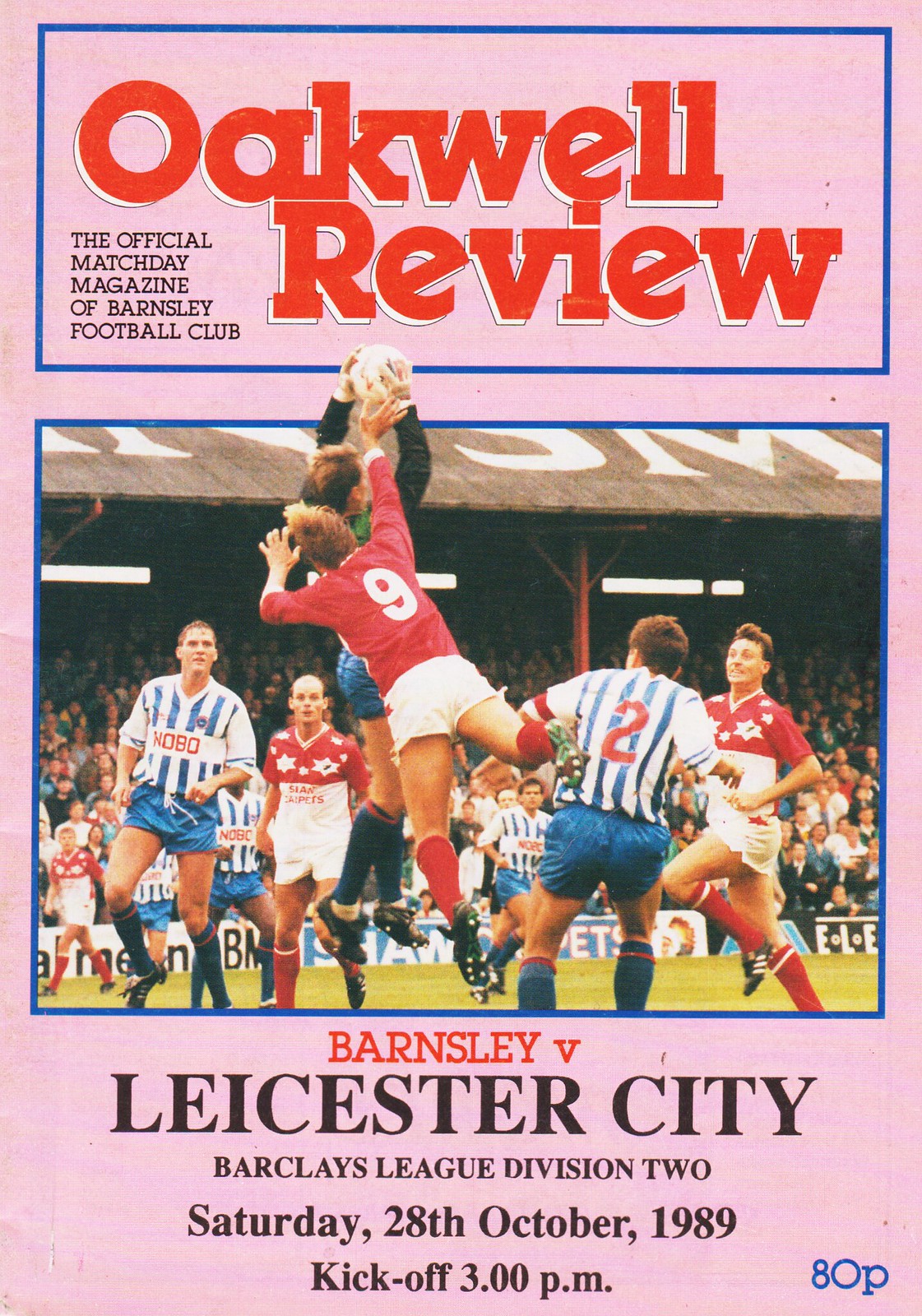On the front cover of a leaflet with a pink background, a blue square at the top contains the title "Oakwell Review" in large red text with a white shadow underneath it. Just below "Oakwell," in the bottom left corner, in small black letters, it says, "The official match day magazine of Barnsley Football Club." Beneath the title section, there is another blue square which houses a dynamic photograph of a soccer match. Central to the image is a player in a red jersey with the number 9 on the back, white shorts, red socks, and black shoes. To his right, there is a player with the number 2 on his jersey, which has white and blue stripes, along with blue shorts and blue socks. Surrounding these central figures are other players in both red and blue jerseys, indicating a game between two teams. In the background, the stadium is filled with spectators, slightly shadowed, though those in the front are lit up. At the bottom of the cover, beneath the photograph, in red text, it reads "Barnsley V." followed by black text "Lycaester City." Below that, it states "Barclays League, Division II, Saturday, October 28, 1989, kickoff, 3 p.m." Lastly, in the bottom right corner, it says "80 pence" (or "ADP") in blue text.